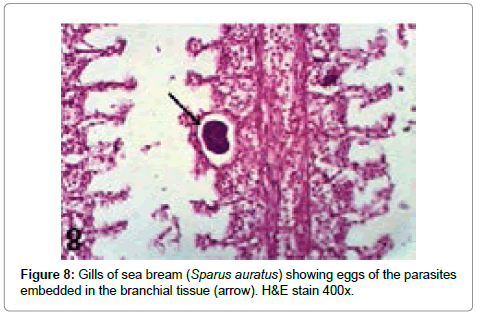This detailed scientific image, likely from a textbook or research paper, is labeled "Figure 8." It shows the gills of sea bream (Sparus aurata) with eggs of parasites embedded in the branchial tissue. The image captures the gills stained with Hematoxylin and Eosin (H&E stain) at a magnification of 400X. The branchial tissue appears light pink with finger-like projections. A distinct, dark purple spherical parasite egg is encased in white on one side of the tissue. A black arrow points toward this parasite egg, highlighting its location. The left side of the image shows more of the pink branchial tissue without eggs. The background is white, suggesting the sample is placed on a glass slide.